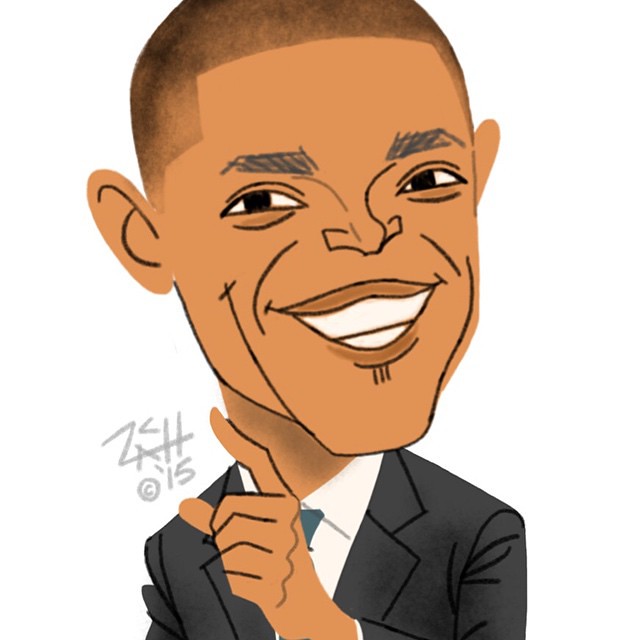This cartoon-style caricature depicts former U.S. President Barack Obama. Set against a plain white background, the drawing features Obama with short, dark hair and light brown skin. His prominent ears, dark eyebrows, and characteristic smile with visible teeth are all accentuated. He is dressed in a grey or black suit, paired with a white shirt and blue tie. His left hand is raised with the index finger pointing outward, while his arm crosses his body, suggesting he is making a point. The caricature artistically exaggerates his distinct features, such as his strong chin, expressive eyes, and broad smile. The drawing is signed by the artist as "Zach © 2015" to the left of Obama's hand.